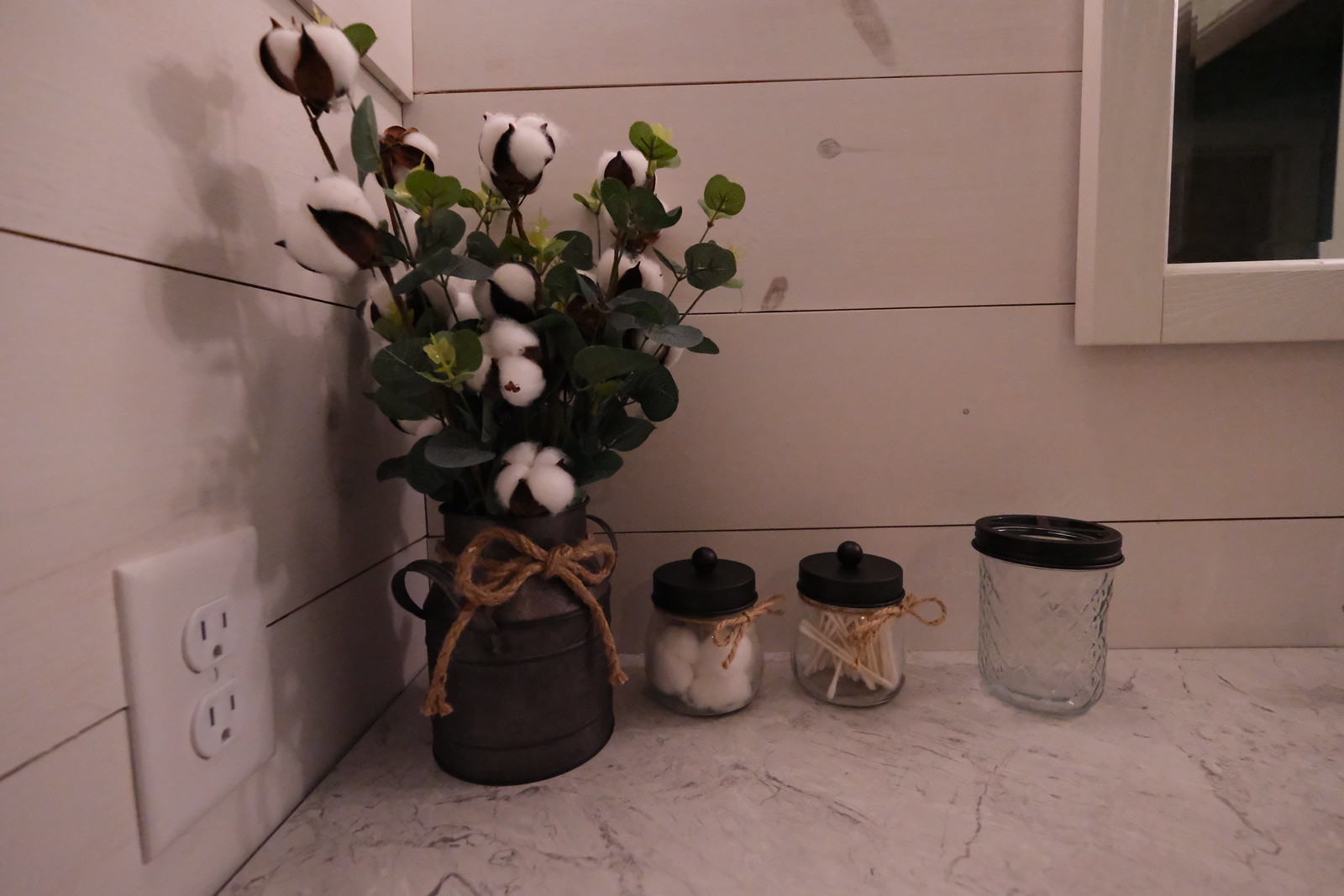This photograph, composed with a slightly darker ambiance, showcases a richly detailed scene centered around a dark metal vase adorned with thick brown rattan string. Emerging from the vase are cotton stems, with the ones on the left reaching higher than the rest. The stems feature puffy cotton tufts and round, deep green leaves. The wall captures the shadow of the vase and cotton, adding depth to the image. 

In the bottom left corner, a white electrical outlet is visible, providing a modern contrast to the rustic setting. To the right of the vase, a collection of smaller jars is arranged. Each jar has a dark lid, with the first two encircled by string. The first jar contains cotton balls, the second houses ear swabs, and the third, a jelly jar, remains empty. 

These items are neatly arranged in a corner atop a white and gray marble surface. The backdrop features whitewashed wooden planks, enhancing the rustic appeal of the scene. The upper right corner of the photograph reveals a framed section of a white mirror, completing this meticulously curated vignette.